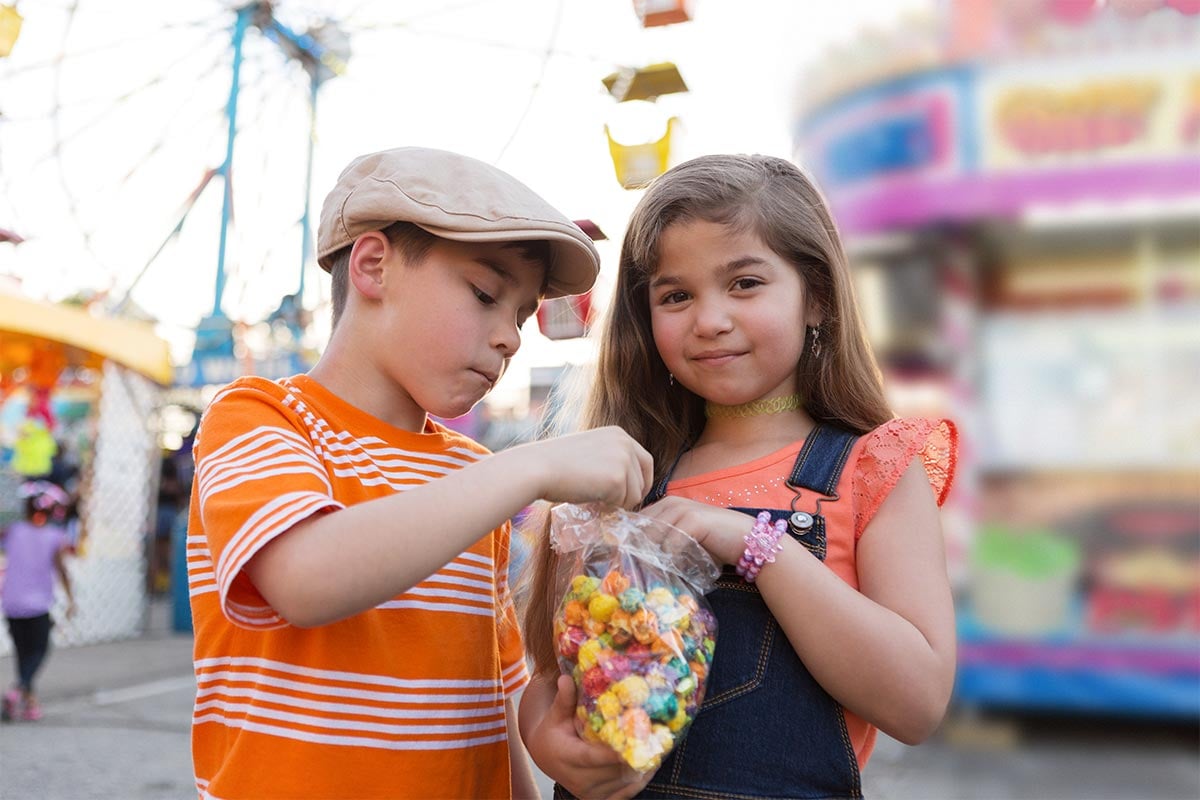In this vibrant, full-color horizontal photograph, we see two young children, a boy and a girl, enjoying a day at a carnival. The background is artistically blurred, hinting at lively carnival scenes, with a Ferris wheel prominently occupying the upper left corner and a colorful food stand on the right. The children, both Caucasian, are central to the image. The boy, dressed in an orange shirt with vertical white stripes and a light tan flat cap, stands on the left. He reaches into a bag of multicolored popcorn, captivated by its contents. Beside him on the right, the girl, wearing blue bib overalls over an orange shirt with frilly shoulders and a neon green choker, gazes directly at the camera, her long brown hair and rosy cheeks adding a touch of charm. A woman in black pants and a blue shirt is seen walking away in the lower left corner, adding to the bustling atmosphere of this carnival scene.